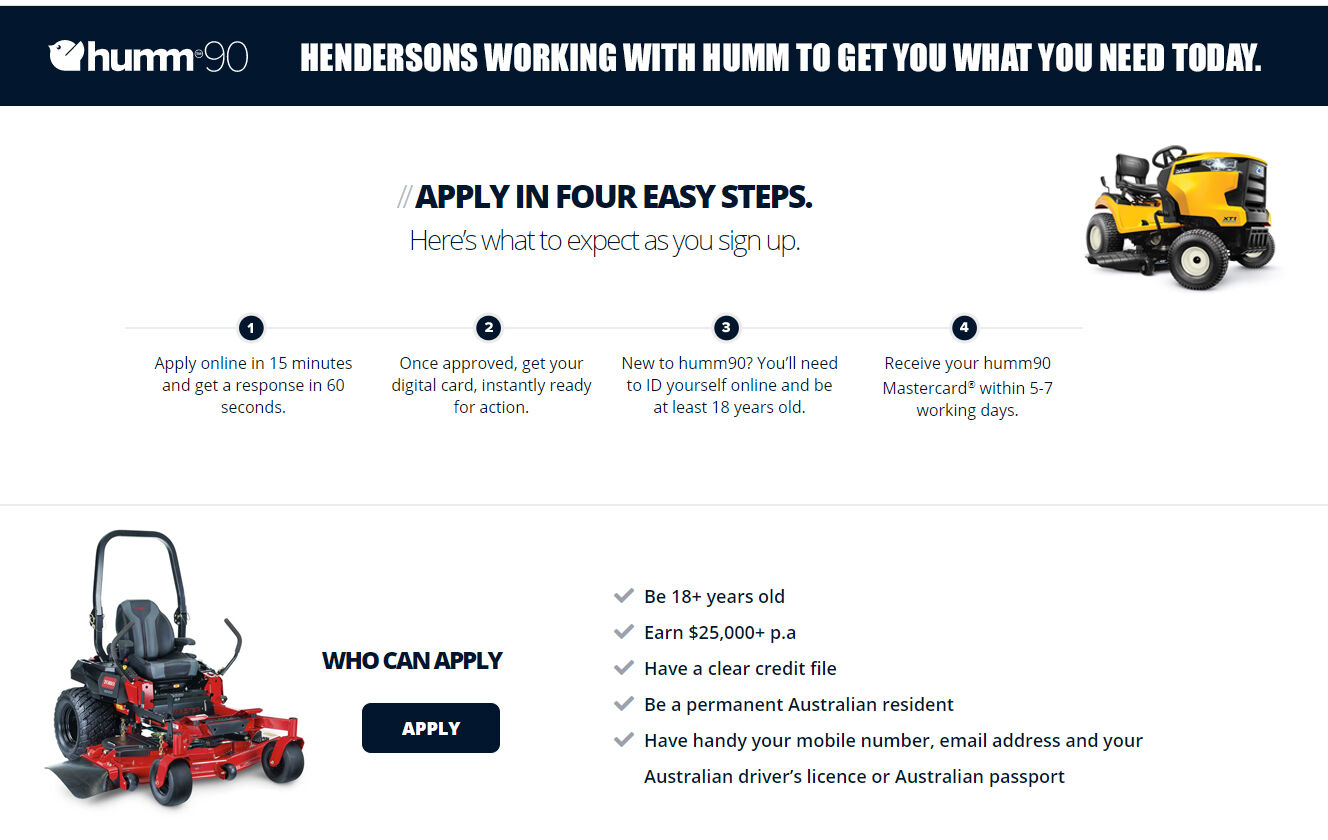The website, titled "Hum90," is presented with a sleek black background. In white text, it states, "Henders working with Hum to get you what you need." Beneath this, the site introduces a section labeled "Apply in four easy steps," explaining the process one can expect when signing up.

In the upper right-hand corner, there is a distinctive image of a yellow riding lawnmower. Below this visual element, a horizontally spread four-part section outlines the application process:

1. **Apply online in 15 minutes and get a response in 16 seconds.**
2. **Once approved, get your digital card instantly ready for action.**
3. **New to Hum90? You'll need to ID yourself online and be at least 18 years old.**
4. **Receive your Hum90 MasterCard within five to seven working days.**

Further down, there is another segment focusing on eligibility. To the left, it features a riding lawnmower with a striking red painted metal body and black components, such as the wheels, controls, and seat.

Adjacent to this image, on the right, the section titled "Who can apply" includes a rectangular, horizontally oriented button with a black background and white text reading "Apply."

To the right of the button, the eligibility criteria are listed vertically with check marks:

- Be 18+ years old
- Earn $25,000 PA
- Have a clear credit file
- Be a permanent Australian resident
- Have handy your mobile number, email address, and your Australian driver's license or Australian passport